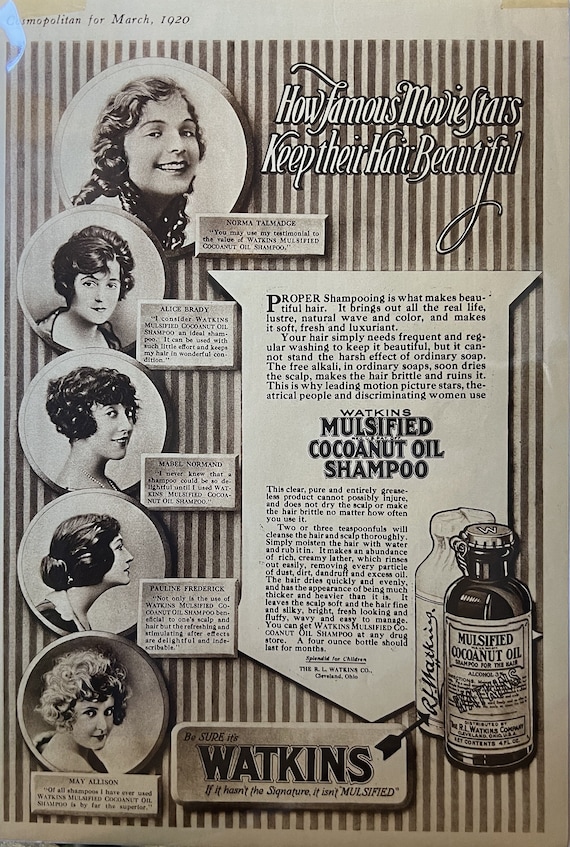This vintage black-and-white advertisement from Cosmopolitan Magazine, March 1920, promotes Watkins Mulsified Coconut Oil Shampoo. The headline, in difficult-to-read white cursive, proclaims, "How famous movie stars keep their hair beautiful." The intricate pinstripe background adds a sophisticated touch but makes the white script challenging to read. The lower part of the poster features a label displaying the product's name and a drawing of the shampoo bottle. Along the left side, five cameo portraits showcase women with elaborately curled hairstyles. These women, identified as movie stars like Norma Talmadge, Alice Brady, Mabel Normand, Pauline Frederick, and Mae Atkinson, each have quotes detailing their positive experiences with the product. On the right side, two or three paragraphs describe the benefits of the coconut oil shampoo, reinforcing its reputation as a film star favorite.